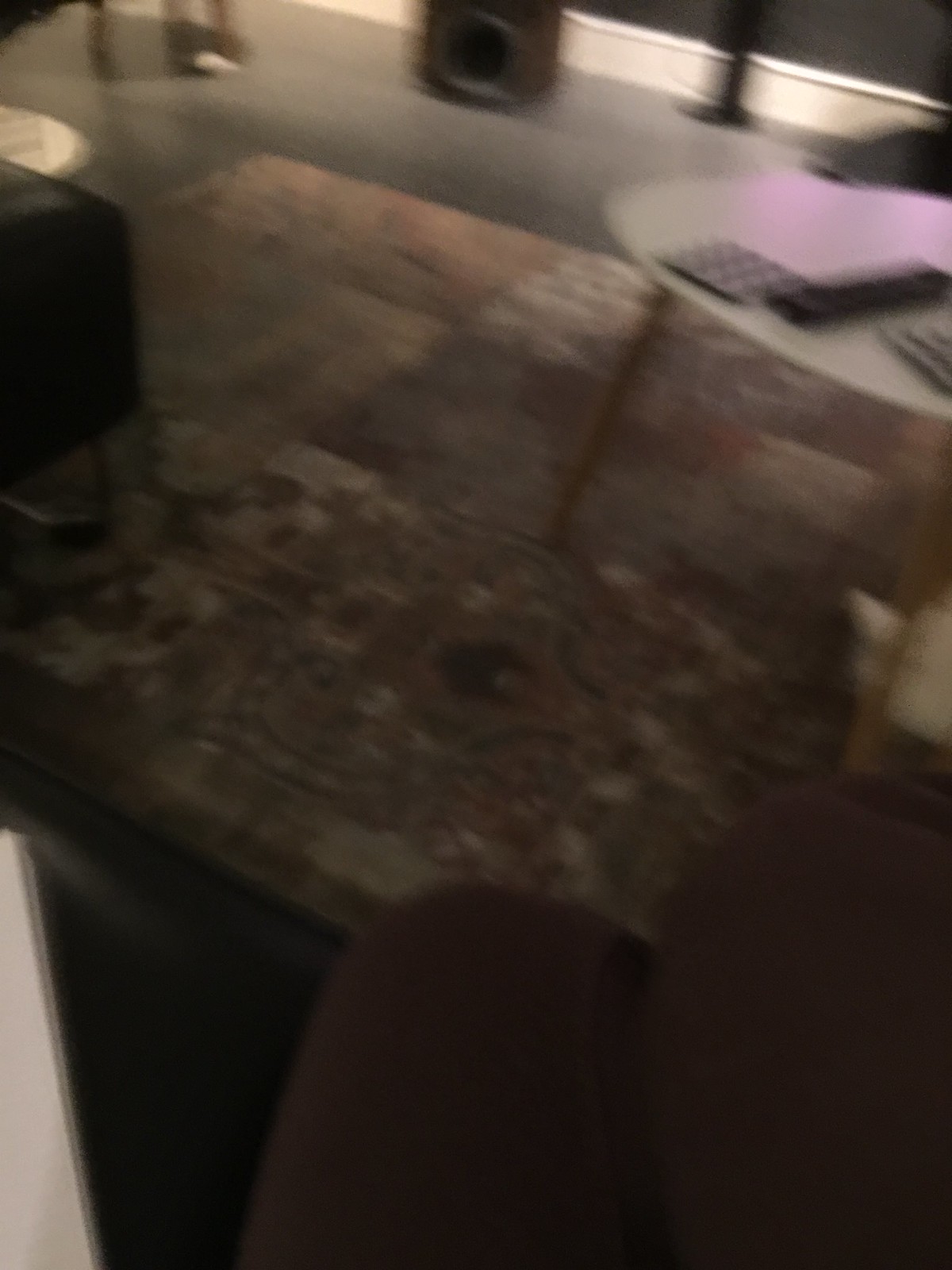This indoor color photograph, taken vertically in a dark and blurry setting, depicts what appears to be a den or living room. The central focus is an area rug displaying an indeterminate pattern in shades of light green, tan, and black. Towards the upper right corner, there is a round white table, distinguished by its thin legs extending into the frame. Adjacent to this table, which features an indistinct pink object on its surface, is a shadow cast by an armchair in the foreground.

The upper left of the image features what might be a credenza or end table, partially visible. A light-tan cushion, potentially part of a two-seat wide sofa or chair, adorned with white stripes and a floral pattern, is positioned centrally. The background showcases white baseboard trim contrasting against dark slate-gray walls, enhancing the dim ambiance. Additionally, a black rectangular speaker and a dark-colored squarish object further add to the complexity of the scene. The photograph is slightly obscured, contributing to the enigmatic quality of this indoor snapshot.